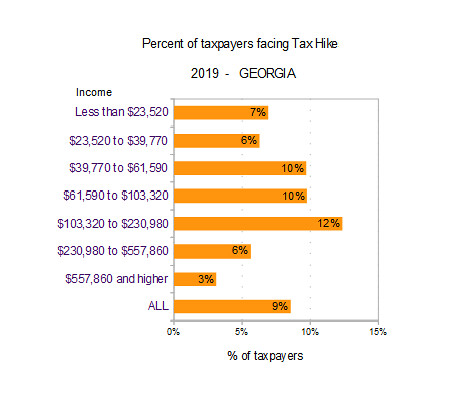The image features a horizontal bar chart prominently centered on a white background. At the top, black text reads, "Percent of Taxpayers Facing Tax Hike, 2019, Georgia." The chart is detailed with various income brackets listed on the left, each associated with distinct percentages: 

- Income less than $23,520: 7%
- Income from $23,520 to $39,770: 6%
- Income from $39,770 to $61,590: 10%
- Income from $61,590 to $103,320: 10%
- Income from $103,320 to $230,980: 12%
- Income from $230,980 to $557,860: 6%
- Income of $557,860 and higher: 3%

There is also a summary percentage at the bottom indicating that 9% of all taxpayers face a tax hike. The chart uses colors white, black, and orange, with text presented clearly across the top, bottom, and left sides of the image, suggesting a design suitable for a government or news website.